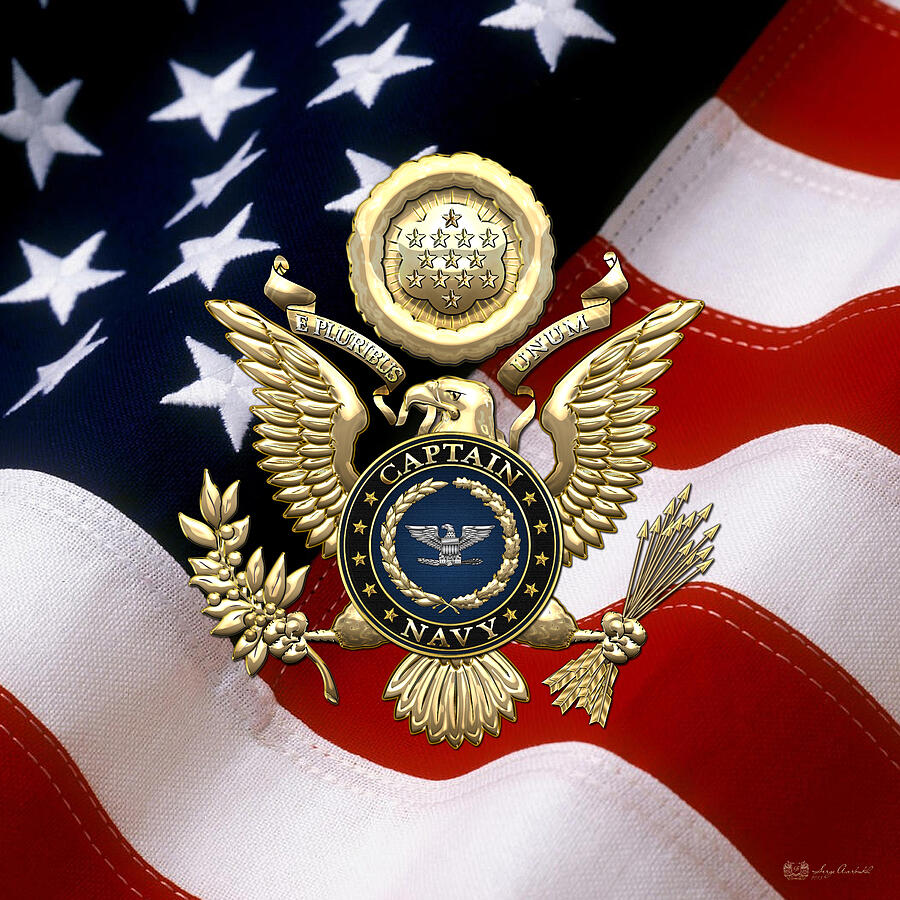This color photograph captures a close-up of an American flag in motion. The composition prominently features a section with white stars on a blue background in the top left, complemented by red and white stripes spanning from the top right to the bottom edges. Central to the image is a detailed gold naval emblem. This emblem showcases a spread-winged eagle looking to the left, clutching an olive branch in one set of talons and a bundle of arrows in the other. The eagle carries a ribbon in its beak inscribed with "E Pluribus Unum." Encircling the eagle is a blue background that reads "Captain Navy" at the top and bottom, flanked by two wreaths. Above the eagle's head, there's a gold circular badge embossed with 13 stars, further highlighted by a metallic gold eagle motif. Small text in the bottom right corner of the image remains illegible. The vivid details and patriotic symbols make this photograph a striking representation of American naval heritage.